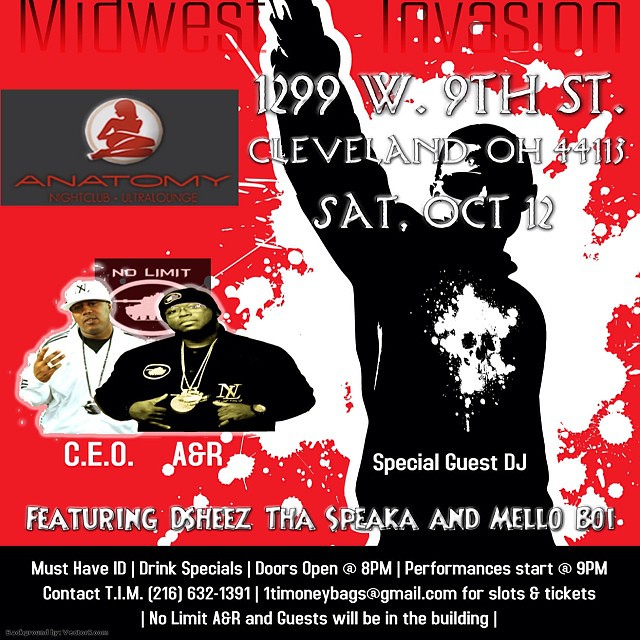The poster for the "Midwest Invasion" event is vividly detailed in striking red, black, and white colors, primarily featuring a vertical design with a prominent red background transitioning to a horizontal black stripe near the bottom. Dominating the top portion of the poster, large black text announces "Midwest Invasion," with key event details outlined below in white: "1299 West 9th Street, Cleveland, Ohio 44113, Saturday, October 12th."

Central to the poster's design is a bold black silhouette of a man with his arm raised, featuring a distinctive cloud skull logo on his chest and wearing sunglasses. Overlaying his head in white text is the event address once more for emphasis.

To the upper left, there's an emblem labeled "Anatomy." This is framed within a circle containing a red silhouette of a woman sitting with her knees drawn up and detailed with red text below it. Two black men are pictured beneath this symbol: one dressed in a white Adidas outfit, chains, and a baseball hat, and the other in a black jacket with chains and an A&R title. They are labeled "CEO" and "A&R," respectively.

The poster also promotes featured artists, listing names like D. Sheez, The Speak Ah, and Mellow We below the special guest DJ. Additional event details noted include a must-have I.D., drink specials, doors opening at 8 p.m., and performances starting at 9 p.m. For tickets and slot information, contact T.I.M. at 216-632-1391 or via email at 1TIMoneybags@gmail.com. The poster also highlights that "No Limit AGR and guests will be in the building."

Overall, the imagery and text provide a comprehensive look into the high-energy branding of this upcoming event.